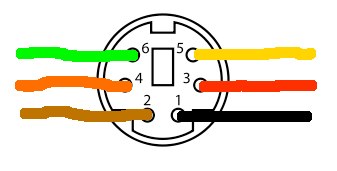The image depicts a black and white diagram with colored wires. The diagram is set against a white background. 

- At the top of the diagram, there's a white circle with a square bump on one side. 
- In the central part of the diagram, there's a rectangle.
- On either side of the rectangle, there are three evenly spaced smaller circles (a total of six small circles).

From bottom to top, the circles are connected by different colored wires:
1. Bottom right circle is connected by a black wire.
2. Bottom left circle is connected by a brown wire.
3. Middle right circle is connected by a red wire.
4. Middle left circle is connected by an orange wire.
5. Top right circle is connected by a yellow wire.
6. Top left circle is connected by a green wire.

The diagram is mainly black and white, with the outline of the device in black and the interior in white. The only colors present are from the six wires, adding a visual guide to the otherwise monochrome image.